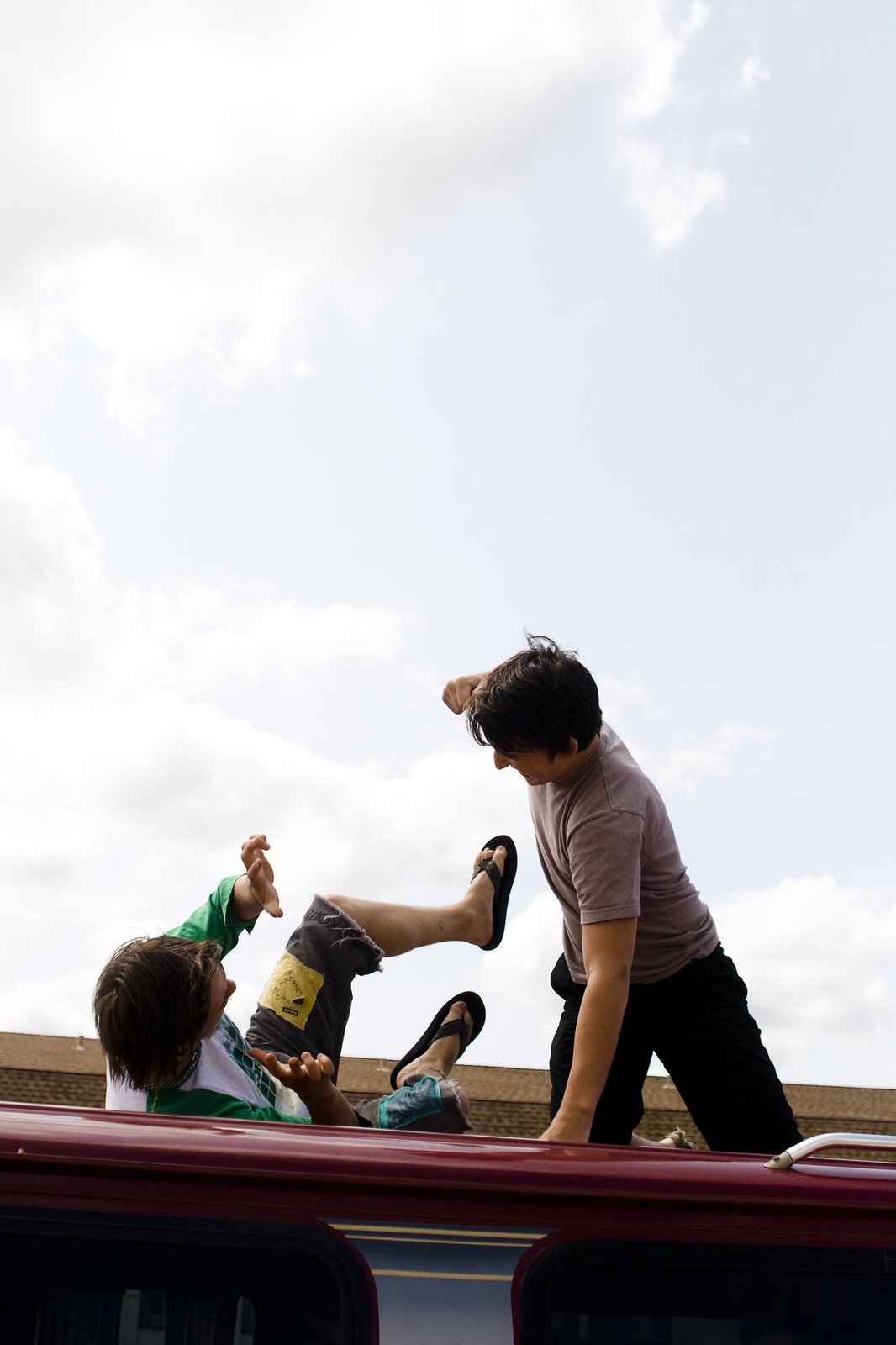In the image, two young men appear to be engaged in a playful scuffle atop a shiny red surface, potentially a vehicle or a boat. The backdrop reveals a bluish-gray sky dotted with white clouds, adding a sense of elevation or openness to the scene. The man on the left lies on his back, legs bent in the air, and hands held up defensively. He is clad in a green and white shirt, brown shorts (or perhaps denim cutoffs), and sandals. His brown hair flows loosely as he gazes to the right where the other man crouches. This second man, with medium-length brown hair, is on his knees wearing a light brown shirt and dark-colored pants. He leans his left hand onto the shiny surface and has his right hand poised in a fist as if about to fake a strike. The red surface they're on features a silver rack at the front right, hinting at a vehicle-like structure. The light-hearted expressions and body language of both men suggest that they are merely horsing around rather than engaged in a serious fight.